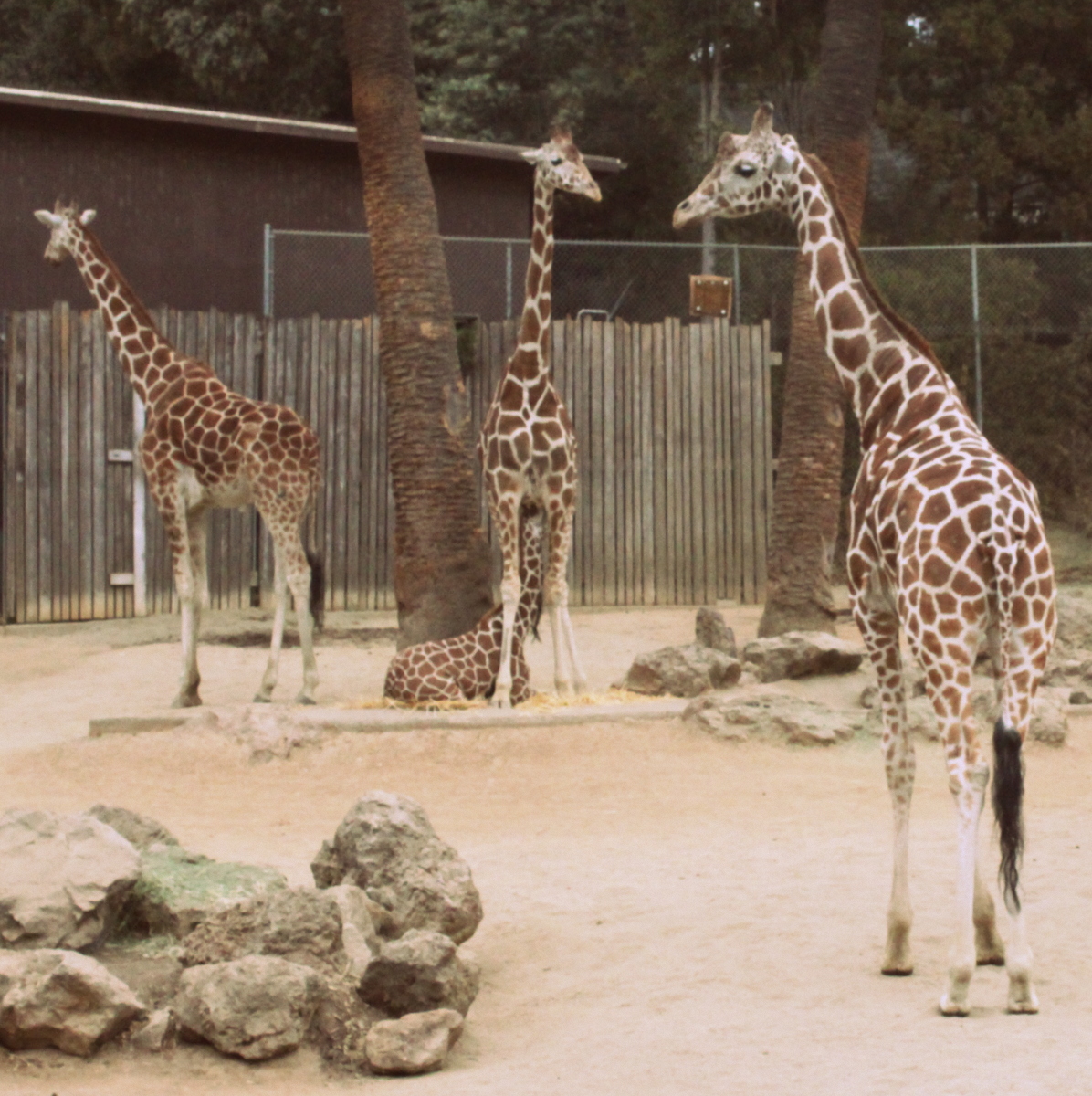In this outdoor daytime photograph set in bright lighting, we observe a habitat, likely at a zoo, showcasing four giraffes. In the foreground to the right, we see a giraffe with its hindquarters facing us, but its head turned left, looking back towards the camera. Centered in the image stand two giraffes; one stands between two tall trees, facing slightly to the right, while beneath it and partially obscured, a baby giraffe appears to be nursing, its neck visible but its head hidden. On the left side, another giraffe is positioned in profile, facing away from the camera. The habitat includes several lumpy rocks in the lower left and center, composed of either granite or sandstone. Behind the giraffes, two tall trees stretch out of frame, while the background features a wooden fence, followed by a higher chain link fence, and a flat-roofed brick building to the left, completing this detailed portrayal of the giraffes' environment.